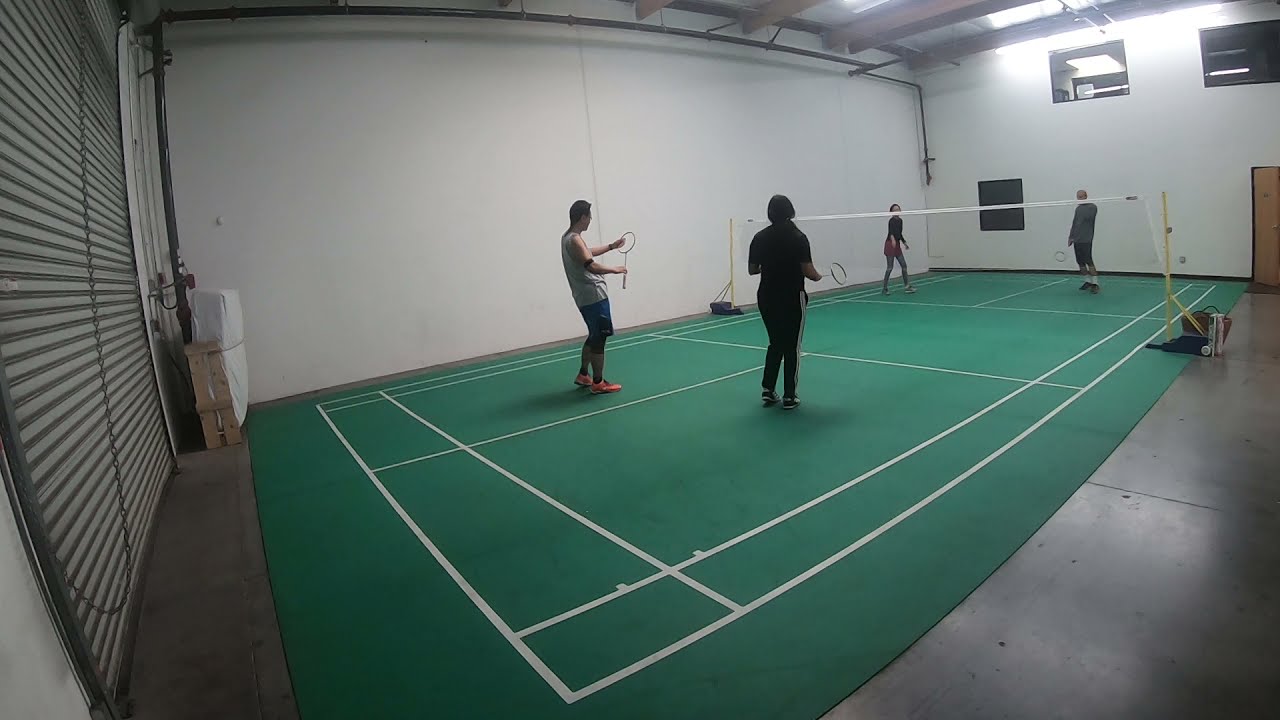In this color photograph of a pickleball court, we see an indoor setting with four players, each occupying a quadrant of the court. The green court is precisely marked with white lines and divided by a net. The players, captured in silhouette, are dressed in athletic attire and holding lightweight rackets. The image is taken from the corner of the court, providing a comprehensive view of the scene. The room's walls are painted an eggshell white, and an evident feature is a large, closed corrugated aluminum garage door on the left. Overhead, exposed beams and lighting fixtures hang from the ceiling, illuminating the space that sits above a gray concrete floor. Small windows near the top of the walls hint at the modest size of the gymnasium, adding to the intimate atmosphere of the indoor court.